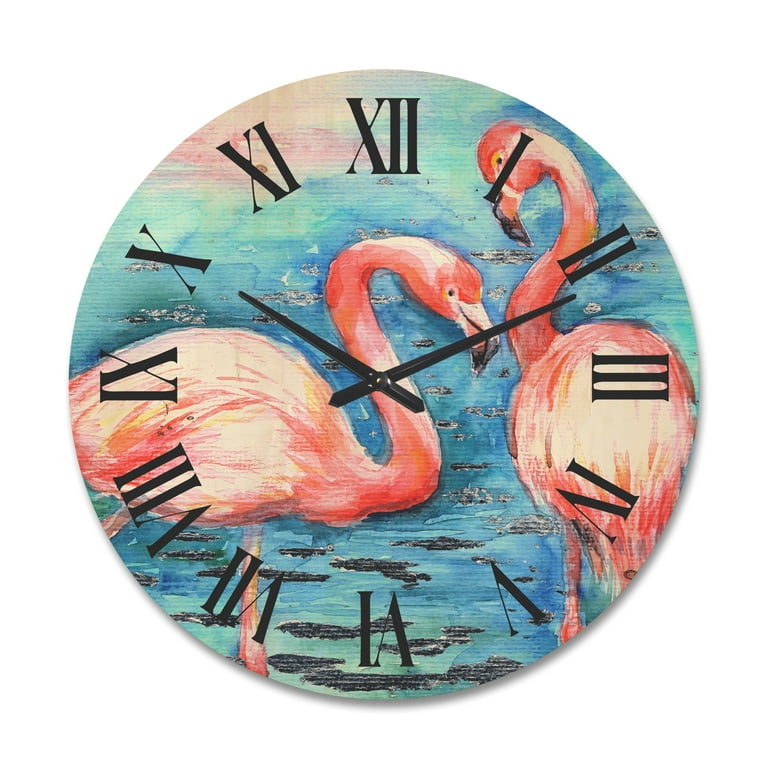The image depicts a round, artistically painted analog wall clock featuring a serene water-themed background with blue hues representing water and dark patches signifying leaves or floating rocks. The clock face is adorned with two elegant pink flamingos. The flamingo on the left, viewed from the side, has its neck gracefully curved as it looks downwards. The flamingo on the right, viewed from the backside, has its neck slightly outstretched and is also looking downward. The flamingos appear to be interacting, with the right flamingo’s beak near the left flamingo's neck. Surrounding this scene are details like green lily pads suggesting they are standing in water. The clock hands are black, with a shorter hour hand and a longer minute hand, and the numbers are depicted in black Roman numerals from I to XII. The time shown is 12 minutes past 10. The overall aesthetic suggests a beach or tropical theme, suitable for a coastal or nautical decor.